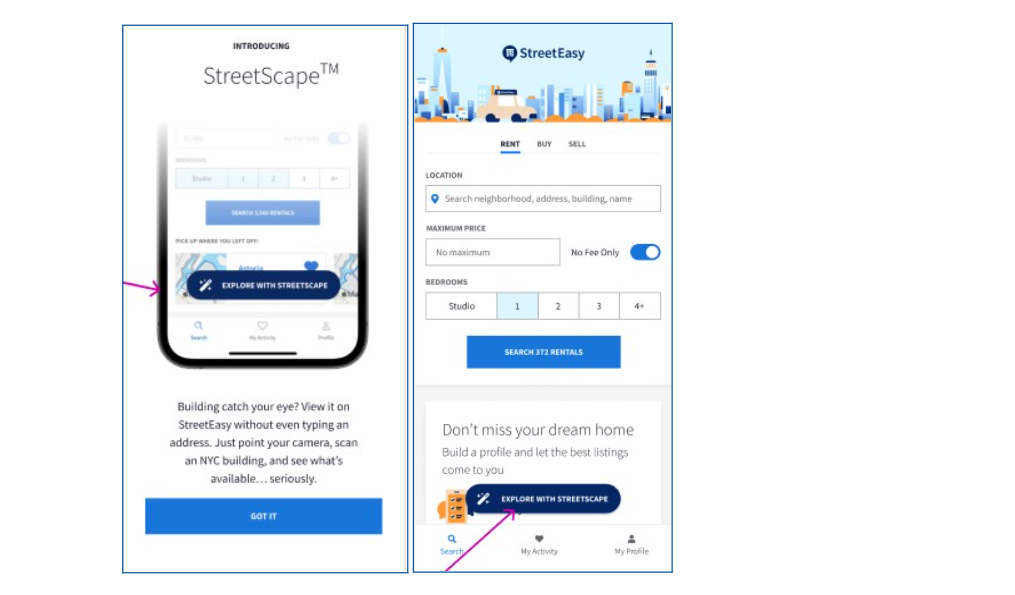Here is a detailed and cleaned-up caption for the given image description:

---

The image consists of two side-by-side screenshots from a mobile app. The screenshot on the left showcases the introduction of a new feature called Streetscape™. It highlights a partial view of a smartphone at the bottom with a blue box overlay that reads, "Exploring with Streetscape." A pink arrow points towards the bottom of the smartphone image. Below this, in gray text, it states, "Building catch your eye? View it on StreetEasy without even typing an address. Just point your camera, scan the NYC building, and see what's available. Seriously." Beneath this text, there's a blue button labeled, "Got it."

The screenshot on the right starts with the StreetEasy logo at the top, followed by a stylized illustration of New York City buildings and a small tan car. Below the illustration, the text reads "Next, Buy and Sell" followed by a gray bar. The interface then provides fields for entering "Location" and "Maximum Price," with an option to toggle "no fee only" listings. Users can select the number of bedrooms they desire, ranging from Studio to 4+. Below these options, there's a prompt to "Search Rentals" (the middle word is unclear), and a white box encouraging users to create a profile with the text, "Don't miss your dream home, build a profile and let the best things come to you." Additionally, there is a blue button labeled, "Explore with Streetscape," emphasized by a pink arrow pointing towards it. At the very bottom, navigation options are displayed: "Search," "My Activity," and "My Profile."

---

This cleaned-up version provides a clear and detailed description of the elements and layout within the screenshots.